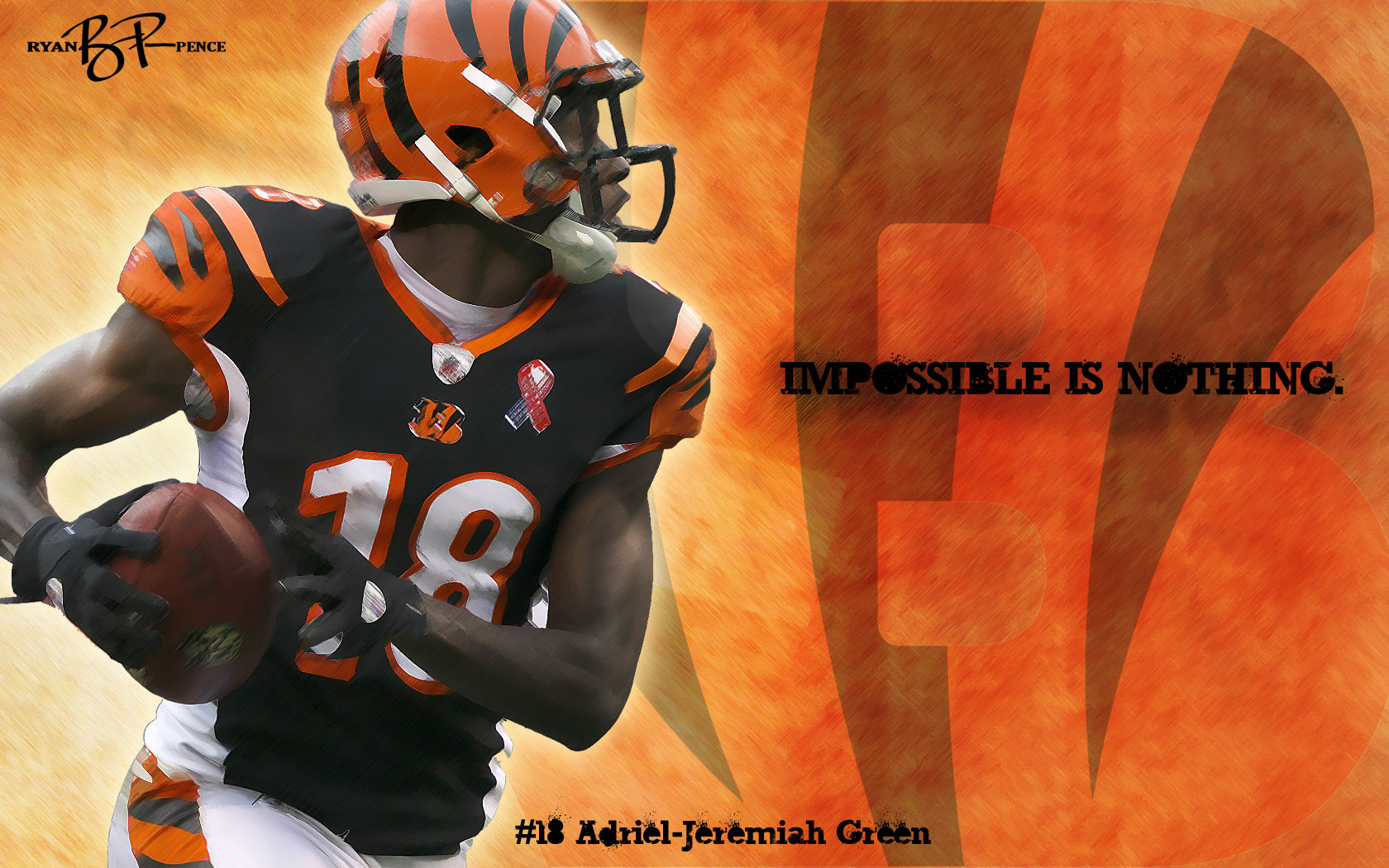The image, a detailed drawing of a football player, features a man in a dynamic pose. Wearing a black and orange uniform with the number 18 prominently displayed in white on his torso, he is holding a football. His right arm is bent with the football clutched in his hand, while his left hand appears to be supporting the ball in front of his body. The player's helmet is orange adorned with black stripes. He dons black gloves and his legs are oriented towards the right, suggesting movement. The background is a blend of orange and black hues, creating a striking contrast. In the upper left corner of the image, the name "Ryan Pence" is inscribed, and in the center of the right side, a bold caption reads, "Impossible is Nothing" in black letters. At the very bottom, the text "Number 18, Adriel Jeremiah Green" is clearly visible, affirming the identity of the player. The scene evokes a sense of action and determination, encapsulating the spirit of the sport.